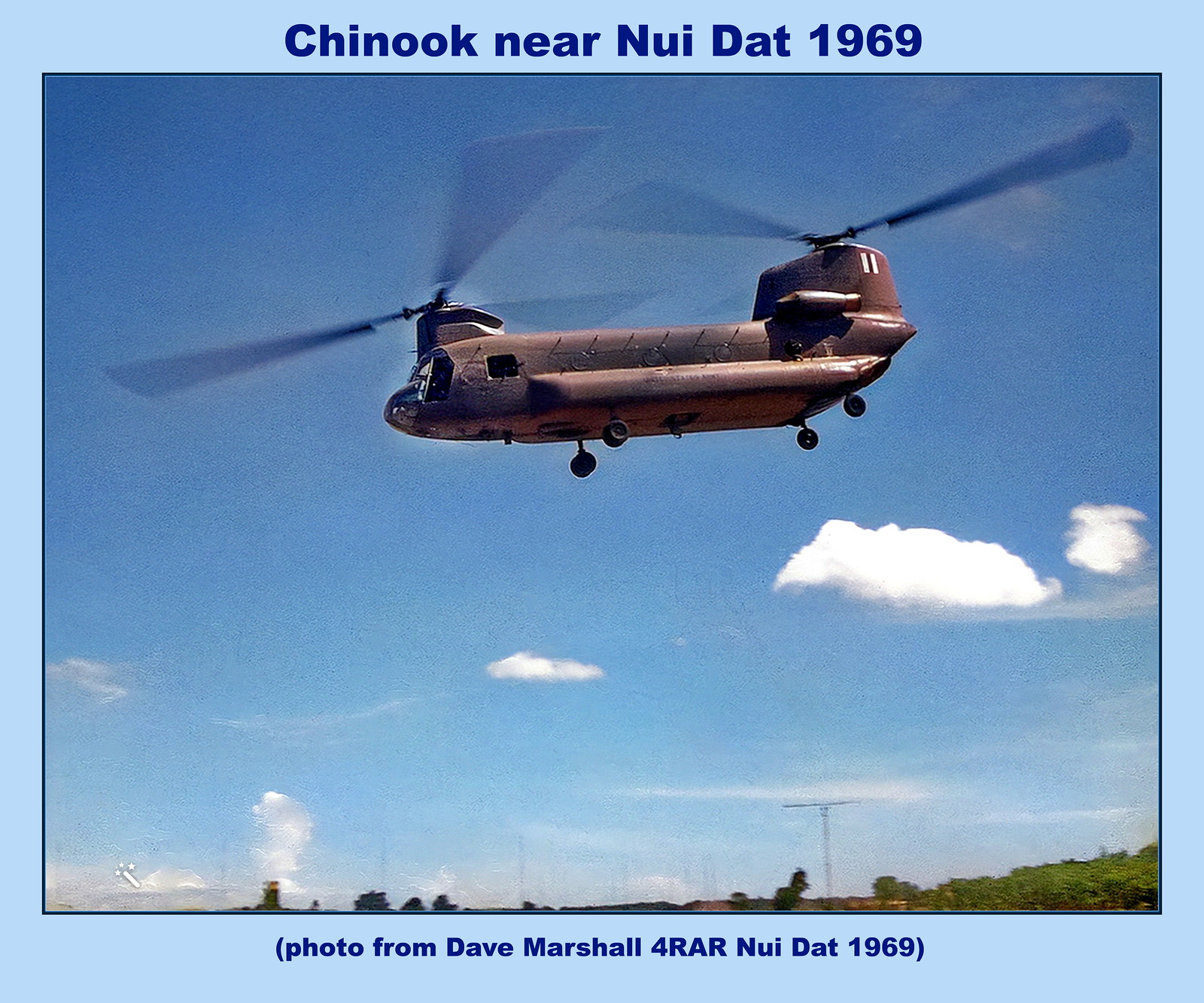The image captures a striking view of a brown Chinook helicopter flying against a backdrop of a clear blue sky, punctuated by one or two billowy white clouds. The helicopter, a long vehicle equipped with rotors on both the front and back, is positioned towards the top of the photograph. In the lower right corner of the photograph, green-covered hills extend to the center of the bottom edge, adding depth and context to the scene. Additionally, there are trees and possibly telephone poles amid the natural landscape below. The picture is framed by a blue border, with text at the top reading "Chinook near Nui Dat 1969" and at the bottom, "Photo from Dave Marshall for RAR Nui Dat 1969." The image combines historical and environmental elements, offering a detailed glimpse into the Chinook helicopter's operational setting during 1969.